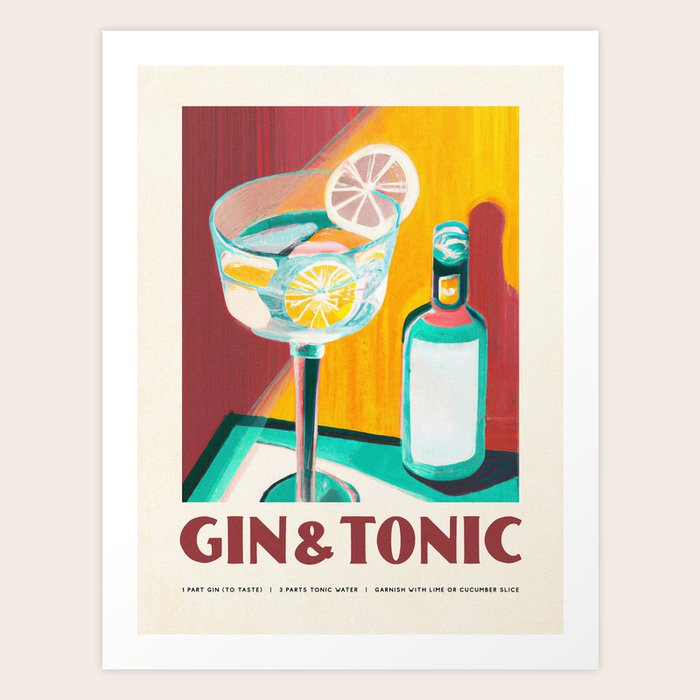The image appears to be a photograph of a vibrant, watercolor painting designed as a poster. It features a light blue wall and a light gray background with a prominently displayed central image bordered by a white frame. The main subject is a detailed illustration of a green glass bottle with a white label and a tall, square-shaped cocktail glass with a long stem. The glass contains a gin and tonic cocktail, depicted with a bluish-green liquid, ice cubes, and slices of citrus fruit, either lime or lemon, with one slice perched on the edge. The background of the painting is a blend of red and yellow shades, adding to the composition's lively character. Beneath the illustration, the title "Gin and Tonic" is written in large red text, followed by a smaller inscription detailing the recipe: one part gin, three parts tonic water, and a garnish of lime or cucumber slices.